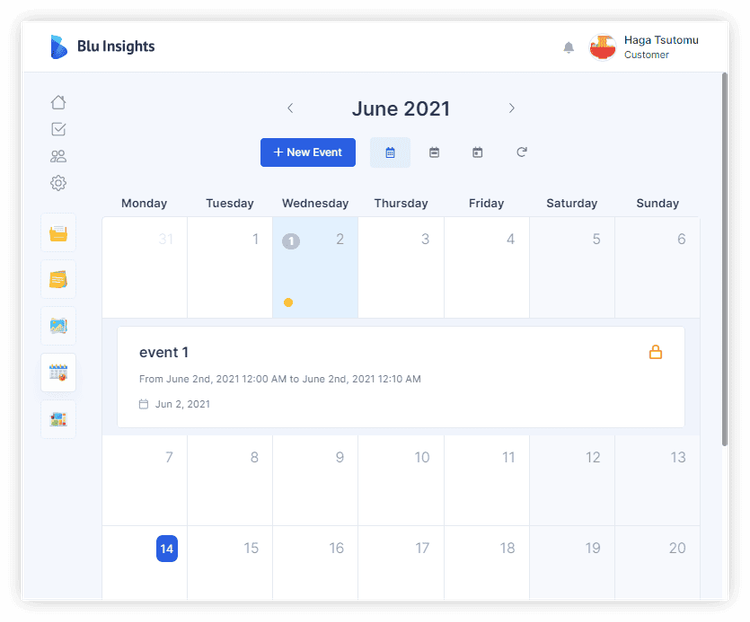The image is a screenshot of a calendar interface from a company named "Blu-Insights" (spelled B-L-U dash I-N-S-I-G-H-T-S). Adjacent to the company name is a stylized "B" symbol that features a gradient color scheme transitioning from blue to turquoise. The calendar is for June 2021.

At the top of the interface, there is a blue "New Event" button, next to which are several icons: two resembling calendars and one that appears to be a forward or redo button.

The calendar layout below this header displays days of the week—Monday, Tuesday, Wednesday, Thursday, Friday, Saturday, and Sunday—starting from May 31 (Monday) to June 6 (Sunday). 

Notably, on June 2nd, a yellow dot and a gray dot are positioned on the left side of the calendar, likely indicating events or reminders. 

In the calendar details, an event labeled "Event One" with a yellow lock icon is set from June 2, 2021, 12:00 a.m. to June 2, 2021, 12:10 a.m. This event’s date is highlighted just below these details. 

Finally, a segment of the calendar shows a range of numbers from 7 to 20, with number 14 highlighted in the same blue color as the "New Event" button, possibly signifying additional significant dates or events.